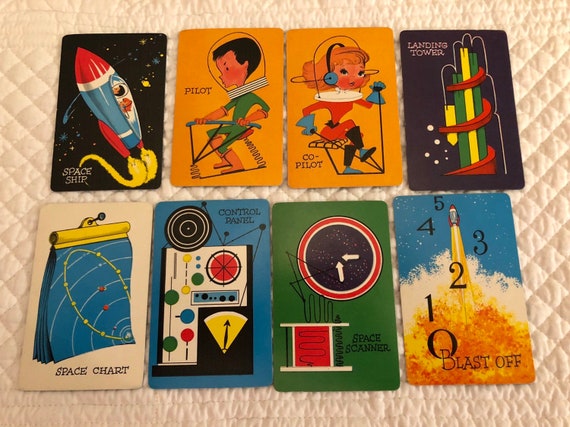On a quilted comforter, appearing a creamy white or pinkish white hue possibly due to lighting, lies a collection of eight vintage toy flashcards arranged in two rows of four. The comforter's quilted pattern adds a textured backdrop to the scene. The cards are rectangular with rounded corners and feature a series of cartoonish, sci-fi-themed illustrations reminiscent of golden age sci-fi. 

The top row starts with a card labeled "spaceship," depicting a blue and red rocket firing its engines amidst a space backdrop. Next is a card labeled "pilot," showing a man in a green astronaut suit and helmet, interacting with a spring-loaded triangle, indicative of spacecraft controls. The third card, "co-pilot," features a young woman with light brown hair, wearing headphones, a red outfit, and a white ring around her neck, similarly interacting with spacecraft controls. The fourth card reads "landing tower," illustrating a towering structure with cylindrical green and yellow sections and a red spiral ramp.

In the bottom row, the first card is labeled "space chart," displaying a notebook with pages showing circular planetary orbits. The next card, "control panel," features a console with colorful buttons and dials. The third card, "space scanner," has a green background with a central black circle surrounded by directional arrows, suggesting the scanning of space. The final card, "blast off," shows a red and blue rocket launching into space, leaving a trail of fiery exhaust, accompanied by a countdown sequence from 5 to 0.

Each card uses vibrant, cartoonish illustrations to teach children about different elements of space exploration, blending educational content with playful, nostalgic design.